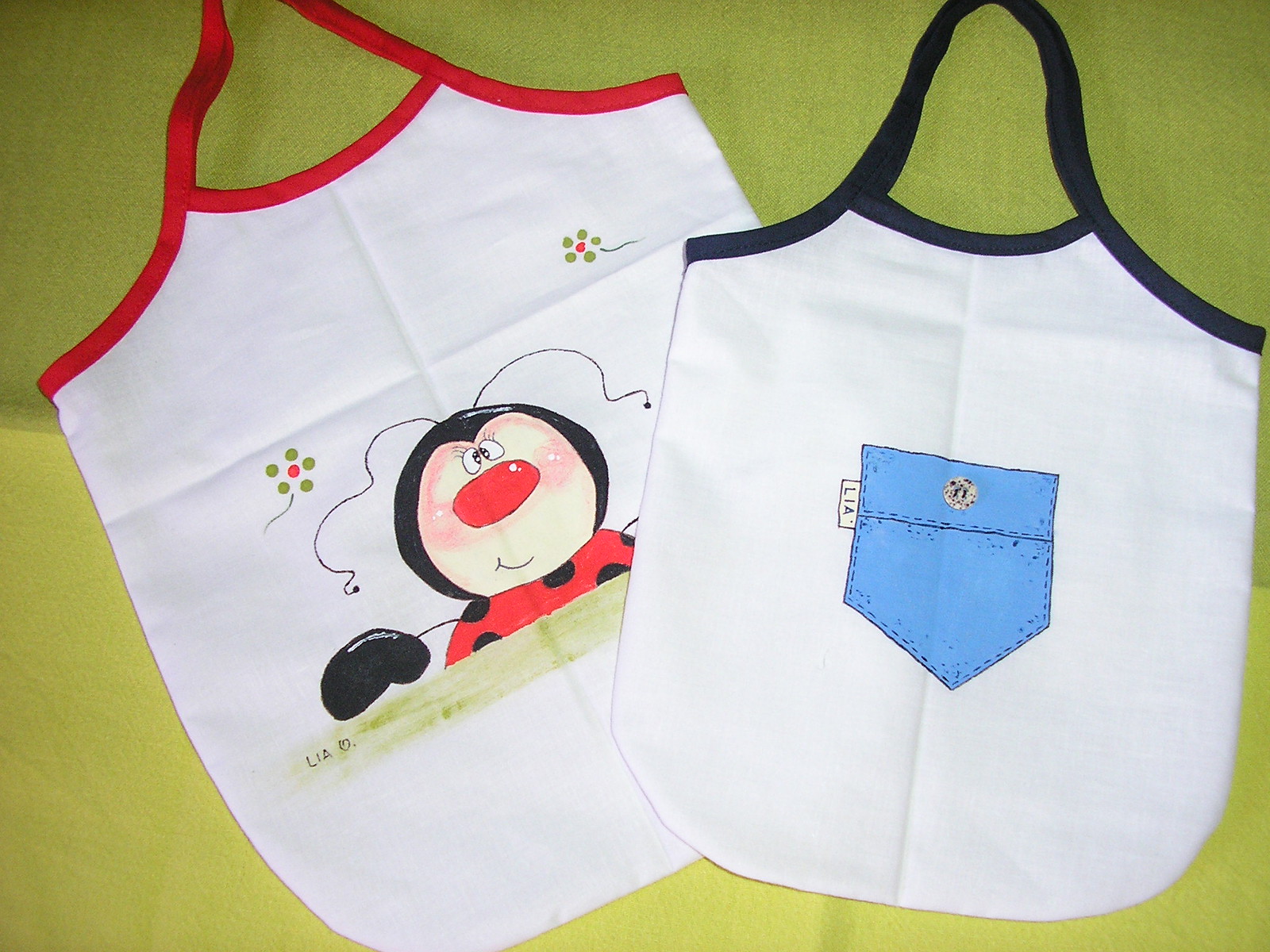This image features two bibs laid out on a light green tablecloth. The bib on the left, positioned slightly tilted, showcases a whimsical design with a cartoon ladybug. The ladybug is red and black with a prominent red nose, two antennae, and sits above light brown dirt. Surrounding it are two whimsical flowers, each with five green petals and red centers, positioned to the top left and right. The bib has red trim around the neck and edges. The name “LIA” is written next to the ladybug.

The bib on the right features a different design, with blue or black trim around the neck. It depicts a blue cartoon pocket that resembles denim, complete with stitching details and a small button at the top. A white tag is visible on its left side. Both bibs display intricate details that make them stand out, such as the flowers and the pocket design. Overall, the setting suggests they're carefully laid out on the table for display or perhaps for a photograph.